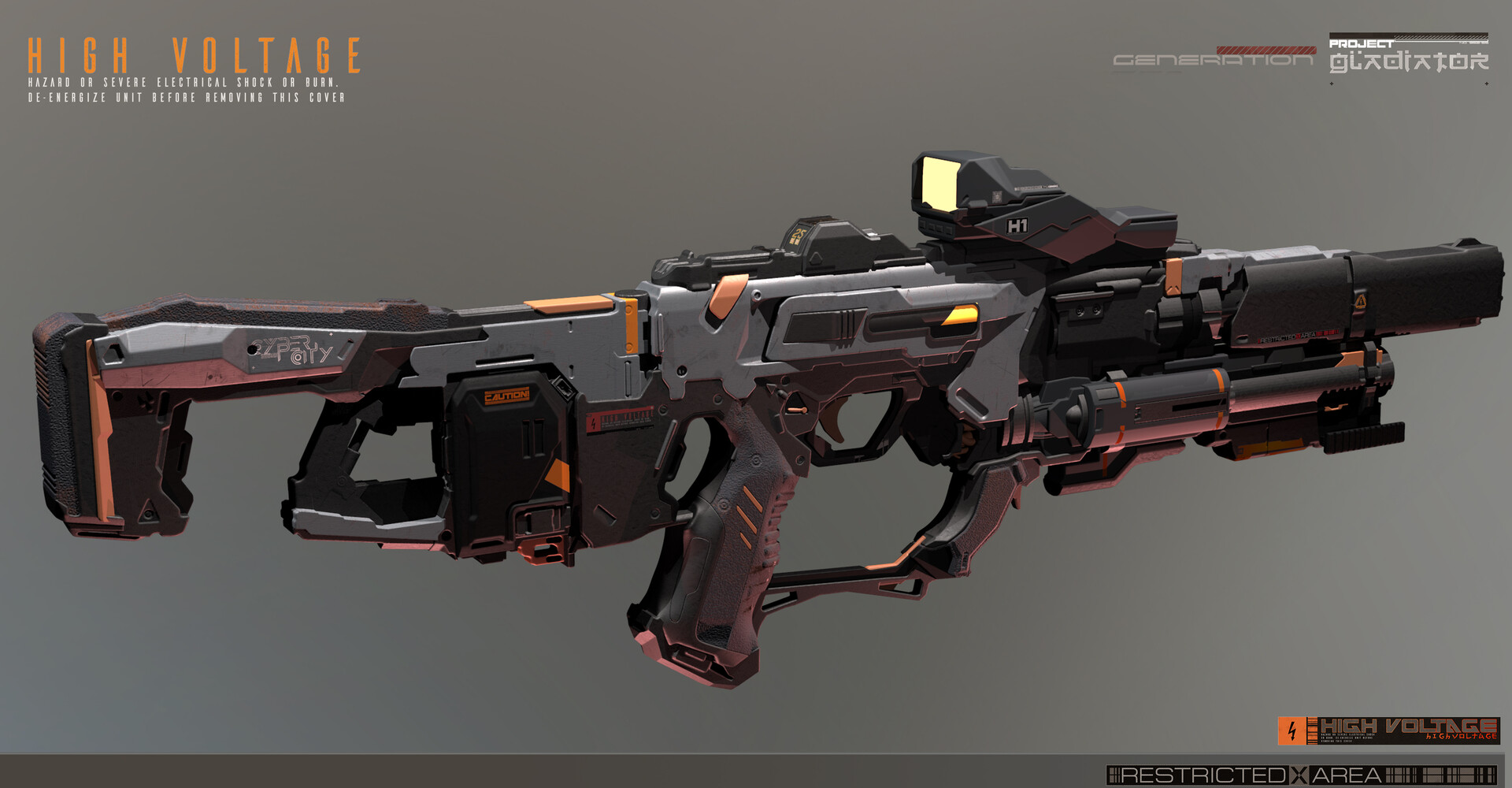This image depicts a highly stylized, futuristic weapon that appears to be a 3D render, likely for a video game. The gun has the exaggerated, over-the-top design typical of cyberpunk aesthetics, featuring a combination of gray and black colors with orange accents. It's a long rifle-style weapon with multiple attachments and pieces, including a glowing scope. The design is distinctly not representative of a real-life firearm, resembling more of a hybrid between a sci-fi gun and something like a nerf or paintball gun. The background is a muted gray, and in the upper right corner, the text "High Voltage" is written in orange. Additionally, smaller, less readable text includes "Project Gladiator," suggesting this could be a prototype or concept model for a game or a creative portfolio piece.